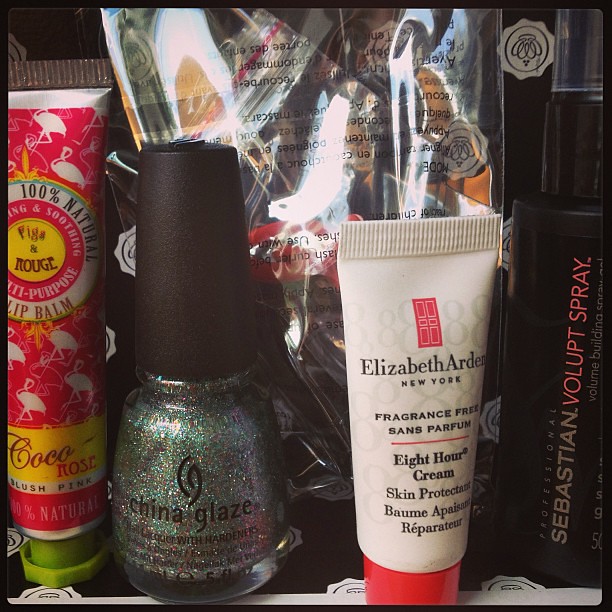This photograph captures a detailed arrangement of cosmetic products, primarily positioned centrally on a black shelf with white trim. Starting from the left, the first item is a tube with a red label featuring white flamingo silhouettes and green cap. It is identified as Figs and Rouge 100% Natural Lip Balm in Coco Rose. Next to it is a bottle of multi-colored glitter nail polish with a black cap, branded as China Glaze. The third item is a small white tube with a red cap labeled Elizabeth Arden New York, Fragrance-Free 8-Hour Cream Skin Protectant. The last item on the right is a black spray bottle with white and red lettering, labeled Sebastian Volup Spray. In the background, there's a glassine bag with some writing on it, reflecting light. The overall setting is a tidy, professional display of beauty products organized in a vertical arrangement on a shelf.